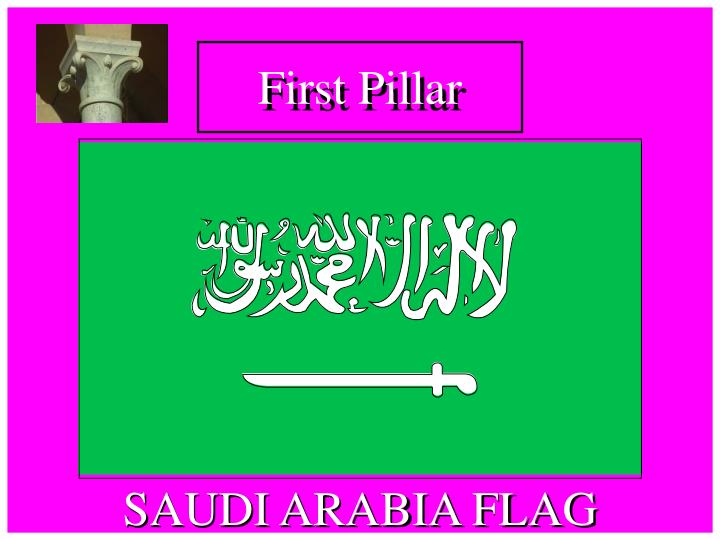The image appears to be a stylized poster with a pink background, featuring various elements arranged in a rectangular format that is wider than it is tall. Dominating the middle of the poster is a green rectangle filled with Arabic text and a white sword, characteristic of the Saudi Arabian flag. Positioned above this green rectangle is the phrase "First Pillar" in white text. To the left of these words is an image of an old Greek-looking column. Beneath the green rectangle, additional white text on the pink background reads "Saudi Arabian flag." The overall layout is divided into three sections: one containing the text "First Pillar" and the column image, one containing the flag itself, and one indicating the flag's identity. The entire composition blends text and imagery, giving an educational or informative feel reminiscent of a PowerPoint slide.